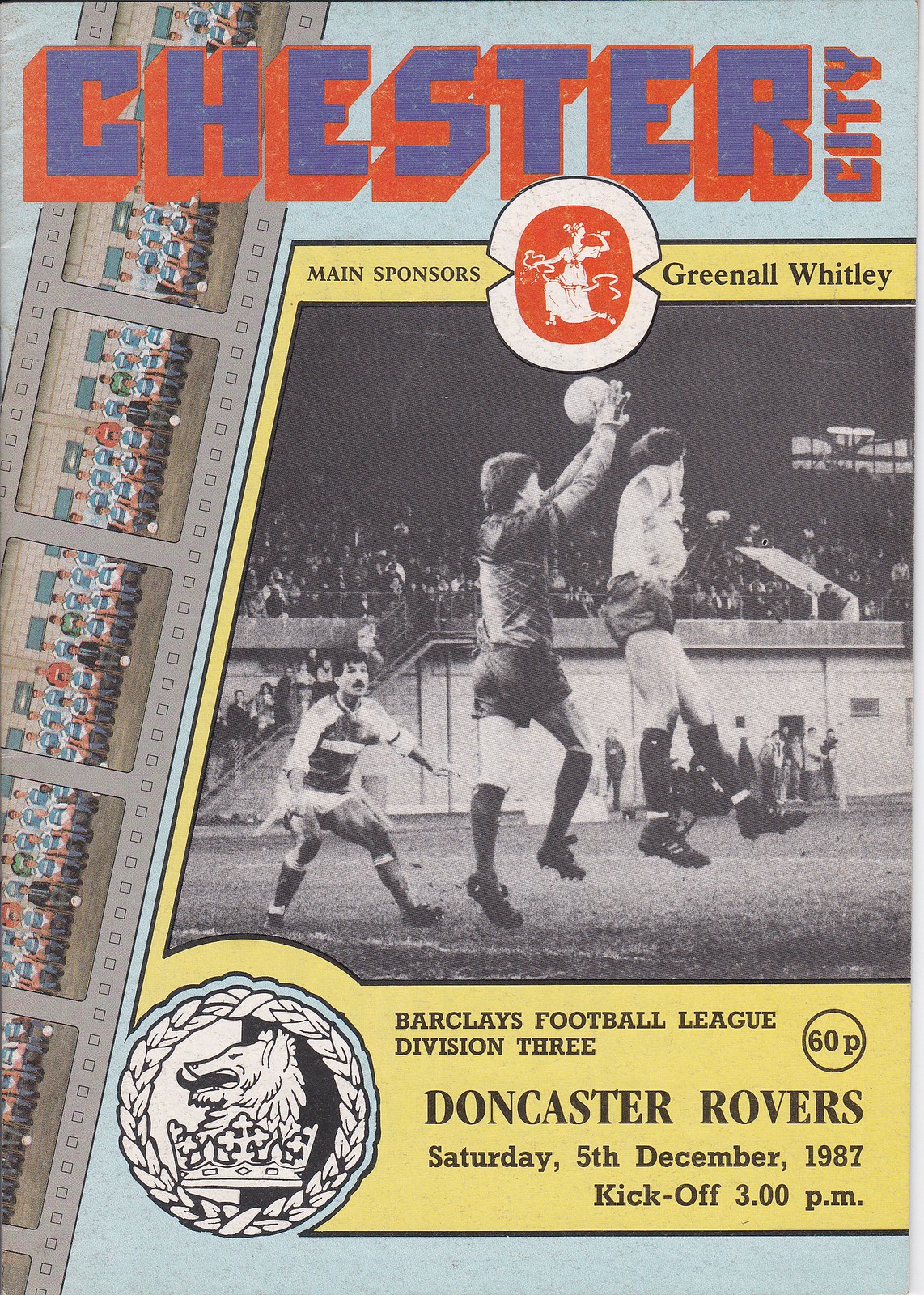The promotional flyer features a light blue background, resembling somewhat crumpled paper. At the very top, in bright blue text with a red background, it reads "Chester City." A tilted film strip runs from slightly right of the top left corner downwards to the bottom left corner. Each panel of the film strip showcases a blue and white uniformed soccer team. 

Centrally positioned is a black and white image capturing multiple players mid-action in a soccer game, framed within a trapezoidal banner. Above this image, in black font on a yellow background, it reads "Main Sponsors: Green Hall, Whitley." 

Below the central image, in black text, details of the event are clearly listed: "Barclays Football League, Division III, Doncaster Rovers, Saturday, 5th December, 1987, kickoff, 3 p.m." The left-hand side of the flyer includes a mascot or icon, resembling a wolf or a lion.